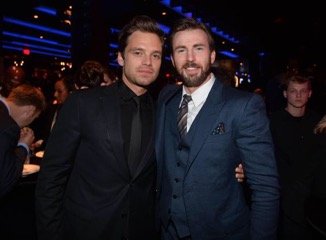In this photo, two men in their 30s are posing elegantly for the camera amid a crowded, formal gathering. Both men have white complexions and short brown hair. The man on the left is dressed in an all-black ensemble consisting of a formal jacket, tie, and shirt, and he sports a goatee. His companion on the right is wearing a navy blue suit, complemented by a vest, a white dress shirt, a striped dark beige tie, and a handkerchief tucked into his pocket. This gentleman also has a beard with a mustache. They are standing closely with their arms around each other, exuding a sense of camaraderie. 

In the background, the setting appears dark, punctuated by the glow of neon blue lights. Among the crowd, a man can be seen eating something, while another looks directly at the camera. The scene suggests a sophisticated atmosphere, possibly within a fancy restaurant, with numerous people standing around tables, adding to the overall lively ambiance.